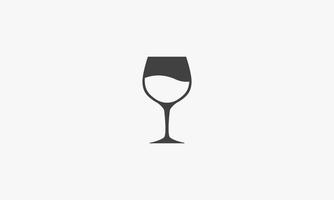The image is a small, rectangular drawing of a wine glass, rendered in black and white on a light blue background. The wine glass is depicted in a simple, digital style, similar to an emoji. The glass is portrayed as half-full, with the top portion shaded in black or dark gray, representing the wine, and the bottom half left white. The wine glass stands centrally in the image, without any surrounding objects or background elements. The overall effect is a clean, minimalist design that highlights the glass itself.